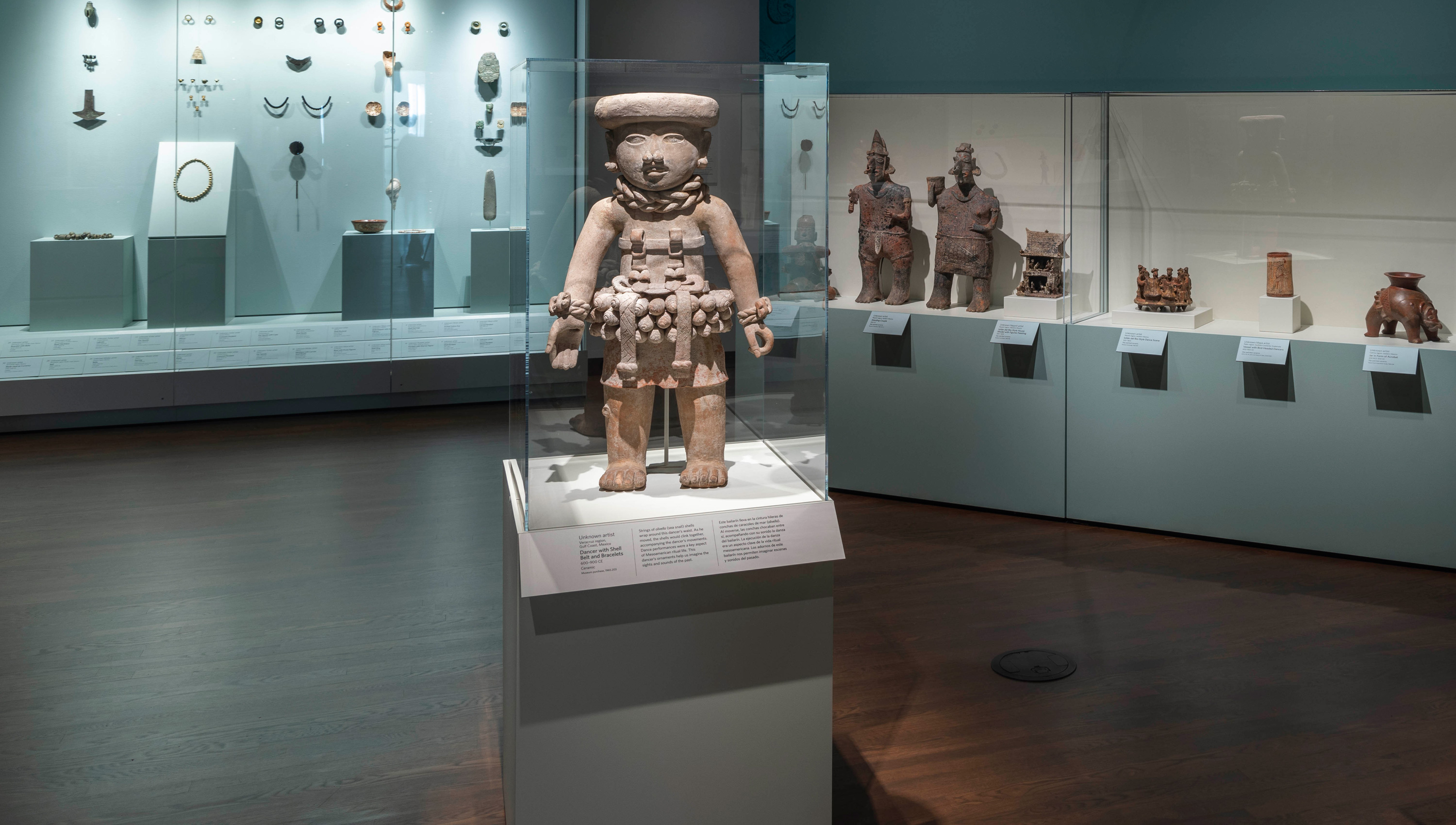This photograph captures an exhibit inside a museum room with a light blue wall and a wooden, brown floor. At the center of the room stands a prominent cuboidal platform featuring a small, ancient-like clay statue of a native man. This statue, housed in a transparent glass casing, portrays a character with human-like features, dressed in peculiar attire including a skirt adorned with circular shell beads or nuts, a rope-like necklace, and a distinctive flat headwear. Surrounding this central display, dispersed near the walls, are additional glass-encased shelves showcasing various other ancient statues and artifacts. Small informative plaques accompany these artifacts, though the text is too fine to read from this vantage. The room's subtle yet intricate arrangement of old sculptures and artifacts, along with the earthy and neutral color palette comprising browns, blues, whites, and blacks, evokes the ambiance of a meticulously curated museum exhibit, perhaps dedicated to tribal or rainforest cultures.